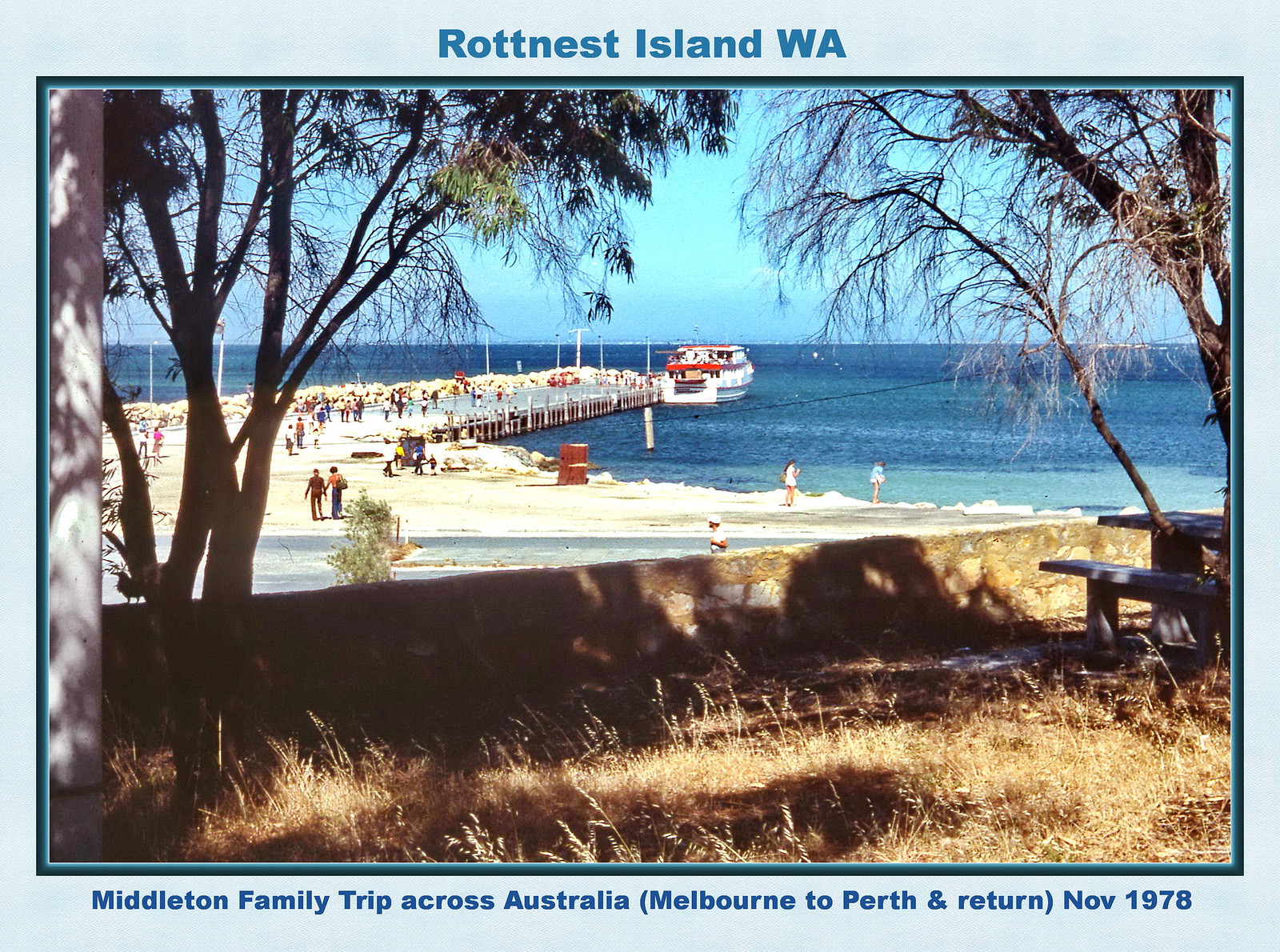This color photograph captures a serene coastal scene at Rottnest Island, Western Australia, during the Middleton family's trip across Australia in November 1978. In the foreground, a sandy beach stretches along the shoreline, leading to a wooden pier that extends into the tranquil blue waters. At the end of the pier, a white passenger boat with a distinctive red awning is moored. The pier itself is bustling with activity, as both people on the pier and along the shoreline enjoy the picturesque day. The water near the shore is a light, inviting blue, which gradually deepens to a rich, dark blue further out. The photograph is bordered by light blue, with dark blue captions above and below: at the top, "Rottnest Island, WA," and at the bottom, "Middleton family trip across Australia (Melbourne to Perth and return), November 1978."